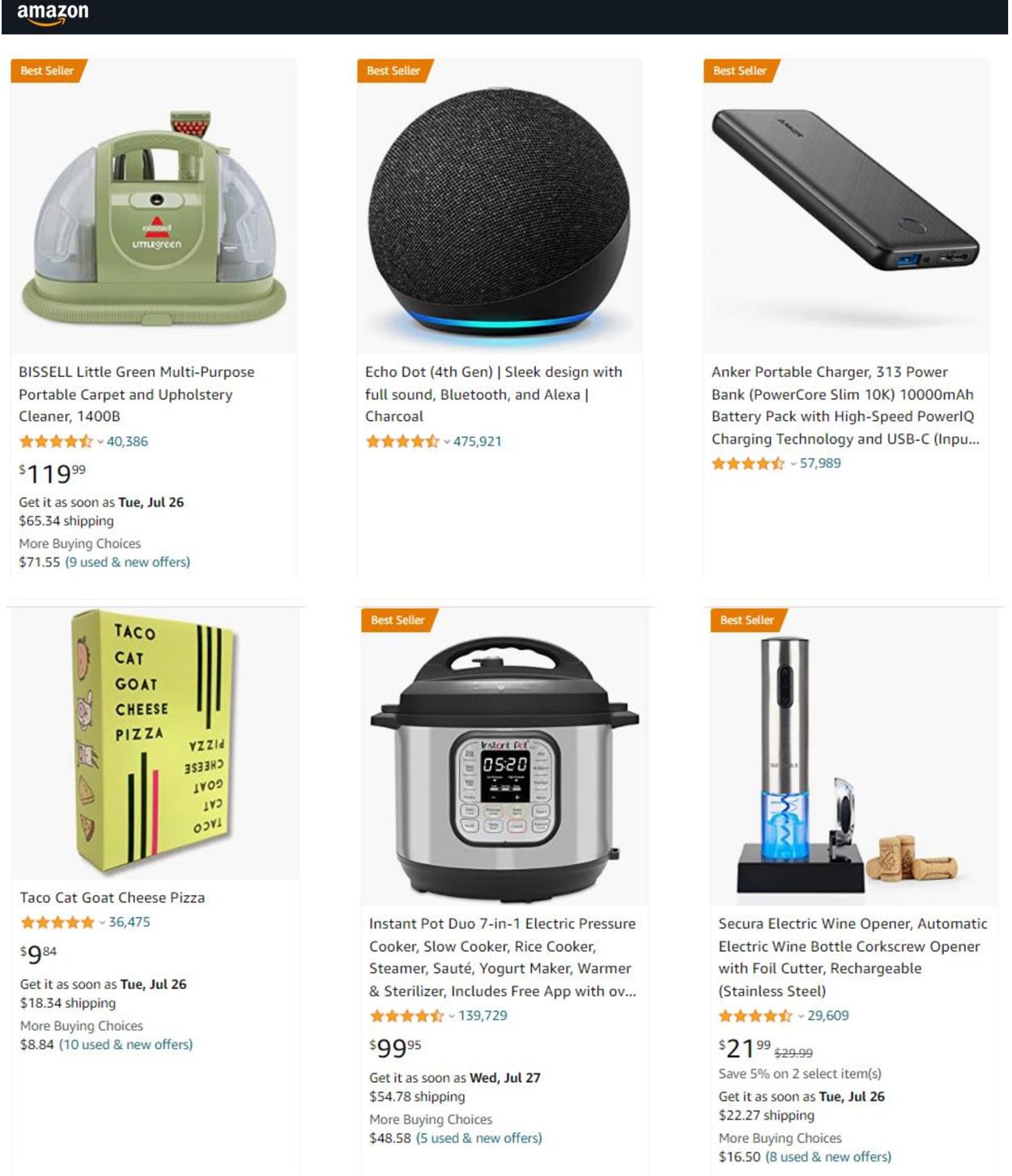The image depicts an Amazon product page, showcasing a variety of top-rated items, all marked with a 'bestseller' badge, except for one. The first row features the Bissell Little Green Multipurpose Portable Carpet and Upholstery Cleaner, followed by the Echo Dot 4th Gen, and the Anker Portable Charger 313 Power Bank. On the second row, there is a single exception to the bestseller status, the Taco Cat Goat Cheese Pizza, packaged in a green box with black printing. Next to it, the image shows the Instant Pot Duo 7-in-1 Electric Pressure Cooker. The final item in the second row is the Sakura Electric Wine Opener, an automatic device made of stainless steel, complete with a foil cutter and rechargeable capabilities. Small corks are seen lying beside it.